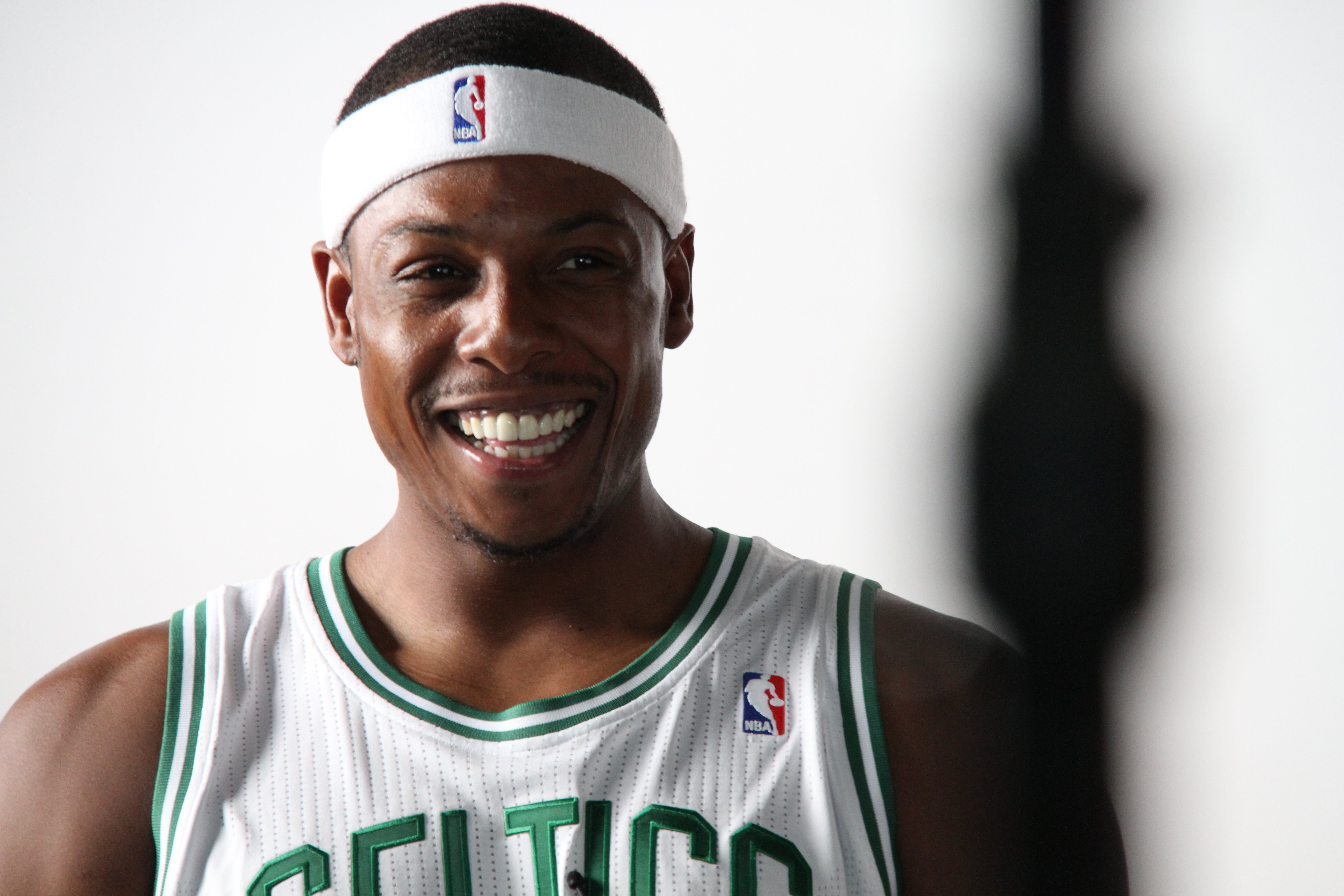This is an older portrait of Paul Pierce, a basketball player for the Celtics, featuring a head-and-shoulders shot. He's wearing a white jersey with green trim that partially reveals the word "Celtics" and an NBA logo, which depicts Jerry West in white on blue and red background. Pierce sports a white headband also adorned with the NBA logo, and his neatly trimmed hair, black mustache, and goatee emphasize his youthful appearance. Pierce, smiling broadly to the point where both his top and bottom teeth are visible, is looking off to the side, adding a candid feel to the image. The background is mostly white, with a blurred black shadow to the right that doesn't obscure our view. His happy demeanor suggests that he might have just achieved something noteworthy on the court.